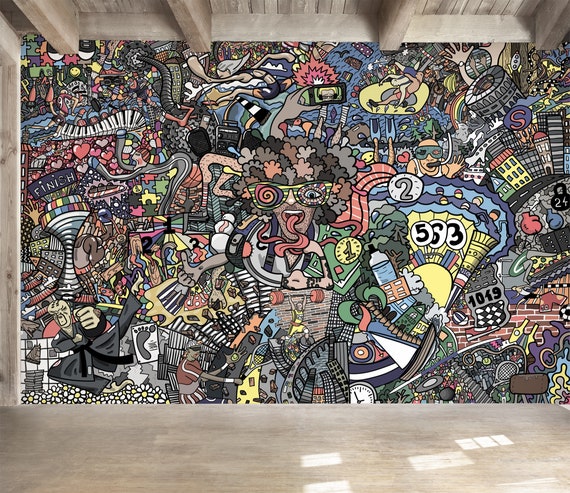The photograph showcases a vibrant and intricately detailed mural located inside a building that appears to be a very clean and well-maintained garage. The spacious interior features a light grayish beige stone floor and is framed by wooden pillars and a wooden ceiling, giving the space a rustic yet refined appearance. 

The mural itself spans from the floor line up to the roof rafters, covering the entirety of the wall. It is a densely packed, colorful graffiti-style masterpiece that blends elements of 3D illustration. The mural is a whimsical collage of characters and scenes reminiscent of a "Where's Waldo" puzzle, with an eclectic mix of figures and objects tightly packed together.

Among the myriad of images, one can spot cartoonish characters such as a man in sunglasses with an exaggeratedly long tongue, wild figures, superheroes, people in motorcycle helmets, and even an iconic depiction of the Roman Colosseum. Additionally, the mural includes an array of diverse elements: people swimming, a piano, animals like rabbits, various buildings, hands, faces, sunsets, race finish lines, keyboards, stones, watch faces, badminton rackets, scuba divers, amusement park rides, and stadium structures. Each element is vividly rendered, inviting viewers to lose themselves in the chaotic yet harmonious scene.

Overall, the mural transforms the garage into a fascinating visual playground, brimming with creativity and artistic flair.